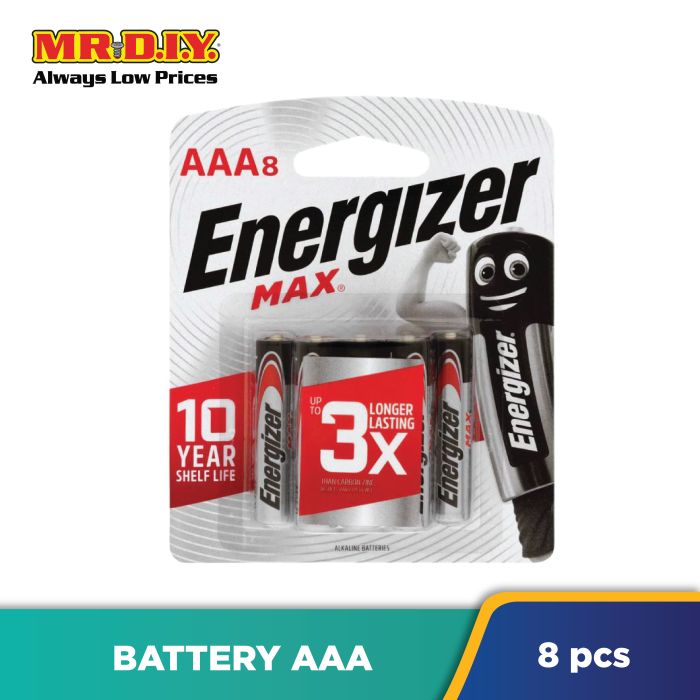Screenshot of an advertisement for Energizer batteries from Mr. DIY. In the top left corner, there's the "Mr. DIY" logo in red text with a yellow background, followed by the tagline "Always Low Prices." Central to the image is a pack of Energizer Max AAA batteries, clearly marked with "10 Years Shelf Life" and "Up to 3 Times Longer Lasting." Beneath the battery pack, there's a teal-colored bar. On the left side of the bar, it reads "Battery AAA," and on the right, inside a small blue box, it specifies "8 PCS," indicating the pack contains eight batteries.